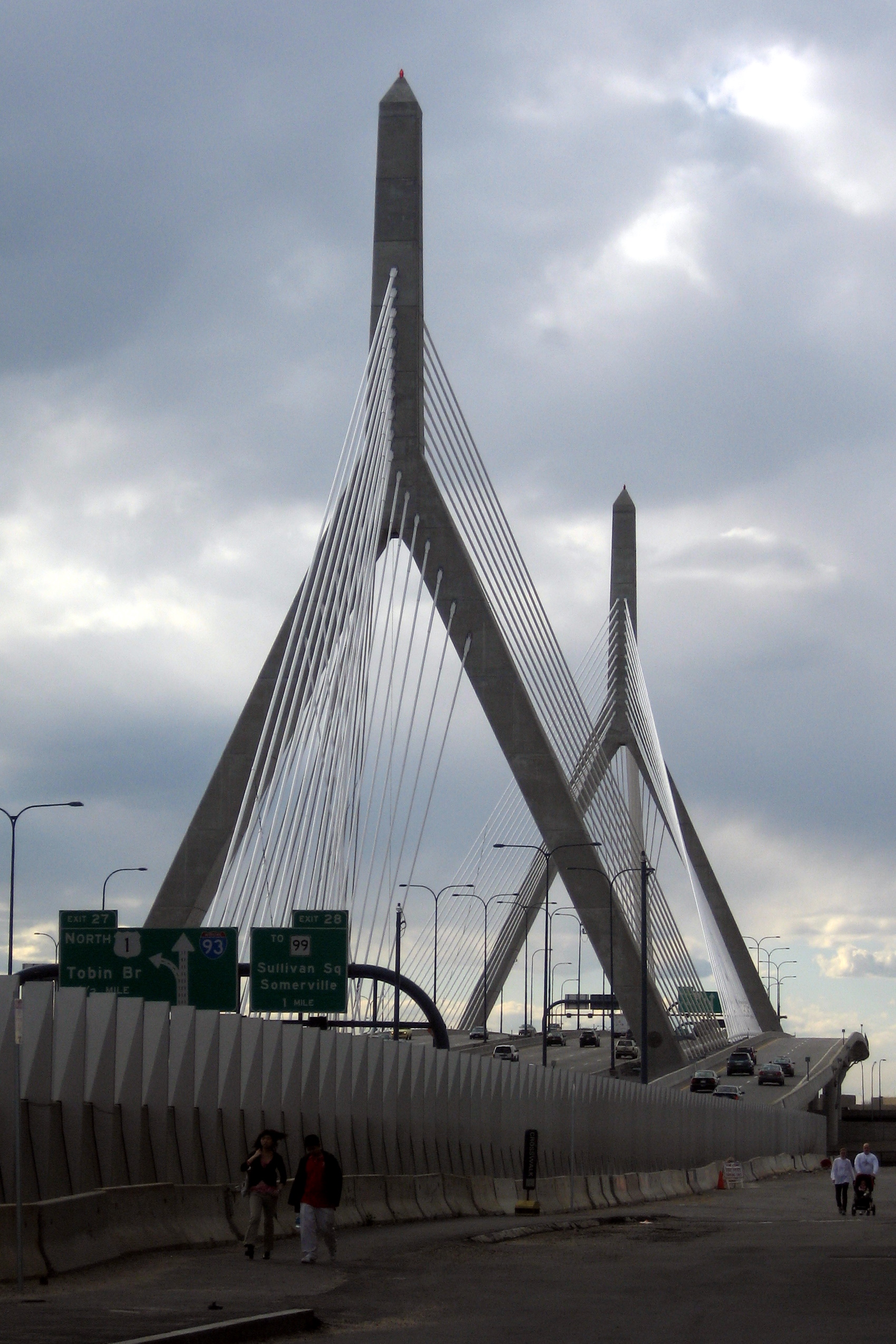The photograph captures a large, multi-lane suspension bridge known as the Tobin Bridge, characterized by its two prominent, wishbone-shaped support pillars. These structures rise dramatically, beginning with a triangular base and extending vertically upwards. The bridge hosts nine lanes: the central five lanes facilitate traffic moving away from the viewer, while the two lanes on either side accommodate vehicles traveling toward the viewer. Below the bridge, there's a gray asphalt parking lot marked with white lines indicating parking spots. Multiple people are seen walking through the parking area; two pairs walk separately, one pair in the foreground wearing black jackets and jeans, and another pair further back in white shirts pushing a baby stroller.

Green and white street signs visible to the left, under the bridge, identify exits 27 and 28, noting destinations such as "Tobin BR," "Sullivan Square," and "Somerville One Mile." The bridge's vertical cables and beams stand out against the overcast sky, adding to the architectural intrigue of this structure. Road barriers define the transition from the parking area to the bridge. The cloudy weather suggests either a dreary day or the approach of evening, adding a somber tone to the scene bustling with traffic and pedestrians.